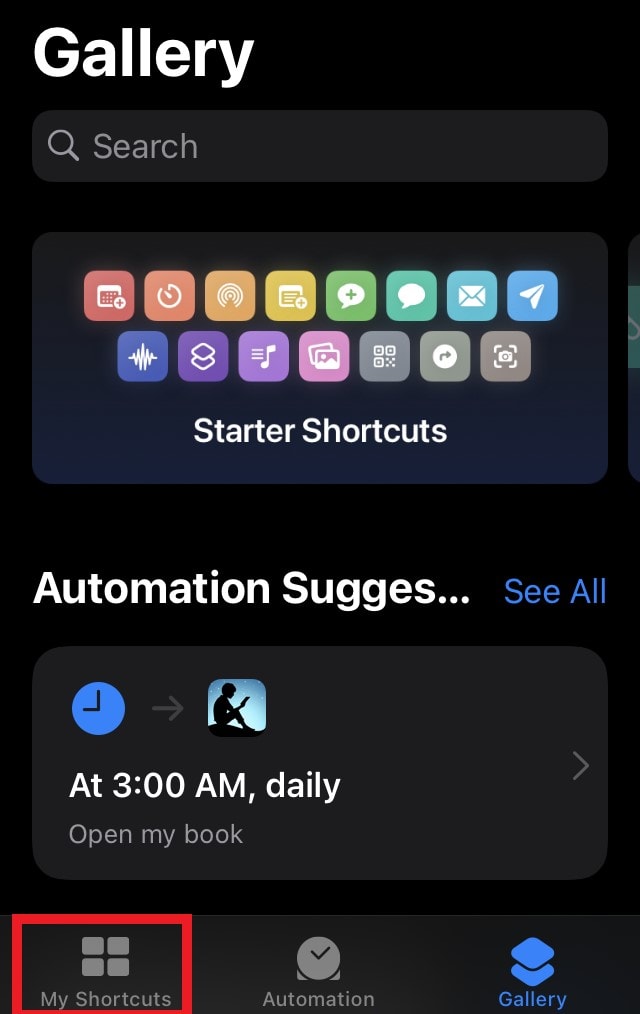The image appears to be a screenshot from a mobile device, potentially a tablet. It features a black background. In the top left corner, "Gallery" is written in white text, followed by a search bar beneath it. Below the search bar is a rounded rectangular area, which has a gradient fading from black at the top to a slightly blue hue at the bottom.

Within this rectangle are two rows of app icons. The top row contains eight icons, and the second row houses seven. The icons are arranged in a rainbow gradient, starting from red on the left and transitioning through green, blue, purple, and finally to greyish-black on the right. Each colorful background hosts a white icon or symbol, including familiar ones like WiFi, messages, email, sound, and possibly a clock.

Beneath these icons, there's a text label reading "Start or Shortcuts," followed by more white text that says "Automation suggests...". To the right, "See All" is highlighted in blue. Below this text, there's a blue clock icon indicating the time is nine o'clock, next to it is a greyed-out arrow. Next to the clock is an image depicting an Amazon Kindle icon, showing a person reading a book against a blue and white background, with the text "At 3 AM daily, open my book" accompanied by a small arrow pointing to the right.

At the very bottom, there are three labels: "My Shortcuts" on the left, encapsulated in a red box that appears superimposed; "Automation" in the center, with icons representing a greyed-out clock; and "Gallery" on the far right, highlighted in blue.